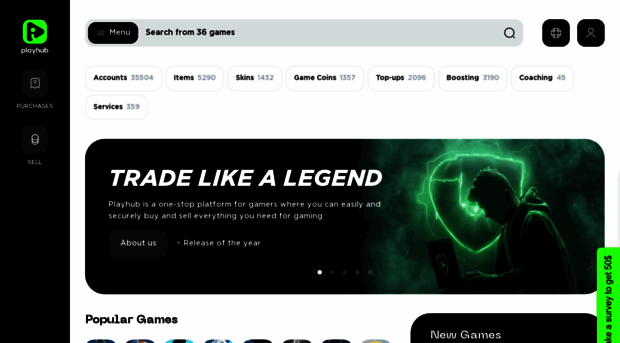This advertisement for PlayHub.com prominently features the website's logo at the top of the screen, alongside bold text reading "Best Free Games" and the URL "playhub.com." Social media icons for Facebook and Twitter are also positioned at the top for easy sharing.

Beneath this header, the text warmly welcomes visitors to PlayHub.com, highlighting the availability of over 11,000 free games suitable for the entire family. These games range from action and sports to Mahjong and bubble shooters, and include a special category for games designed specifically for girls.

The main menu is located just below this introductory text, featuring clickable hyperlinks arranged left to right: Homepage, News, Action, Adventure, Shooting, Fighting, Sports, Strategy, Girls, Racing, and MMO. There is also a magnifying glass icon for search functionality and a three-line menu icon for additional options or settings.

Further down, the "News" section is introduced, offering three articles: "Understanding the Mathematics of Probability in Favorite Games," "Things to Consider When Playing Online Casino Slots," and "The Most Popular Online Casino Games."

Finally, the page lists "Famous Games," showcasing five different selections, followed by another list titled "Best Games," which features eight titles, though none are named specifically.